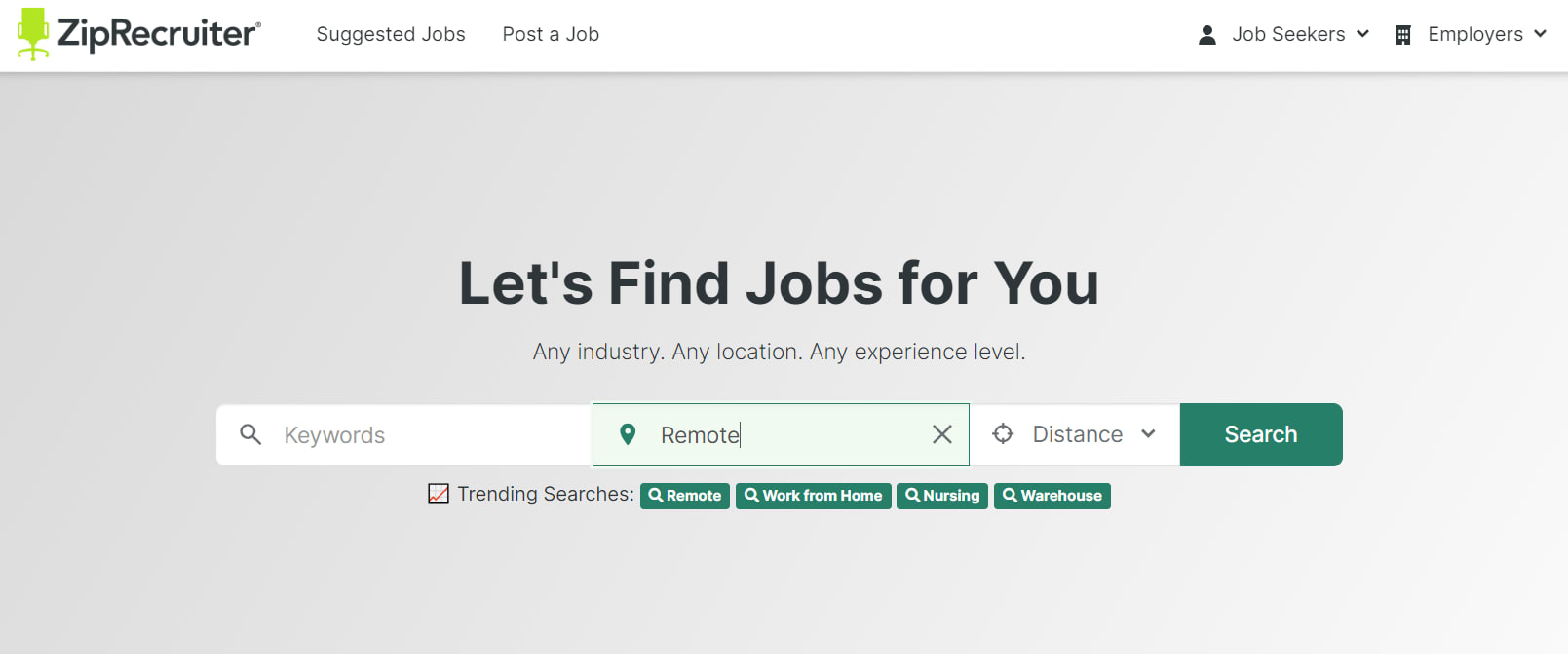The image depicts a screenshot of a webpage from a job search website named ZipRecruiter. Prominently displayed on the left side of the header is a green office chair icon followed by the site's name. The primary navigation menu, extending from left to right, includes options such as "Suggested Jobs," "Post-A-Job," and drop-down menus titled "Job Seekers" and "Employers." The main content area features the headline "Let's find jobs for you," accompanied by the tagline "any industry, any location, any experience level." Below this, there are input fields for job keywords and options to specify remote or local jobs, along with adjustable distance searching parameters. Additionally, the trending searches at the time include "remote," "work from home," "nursing," and "warehouse." The background of the page is gray, contrasting with the green buttons and search bar, which feature white text. This website appears to function similarly to other job search platforms like Indeed or MonsterJobs.com, though ZipRecruiter may not be as widely recognized by some users.